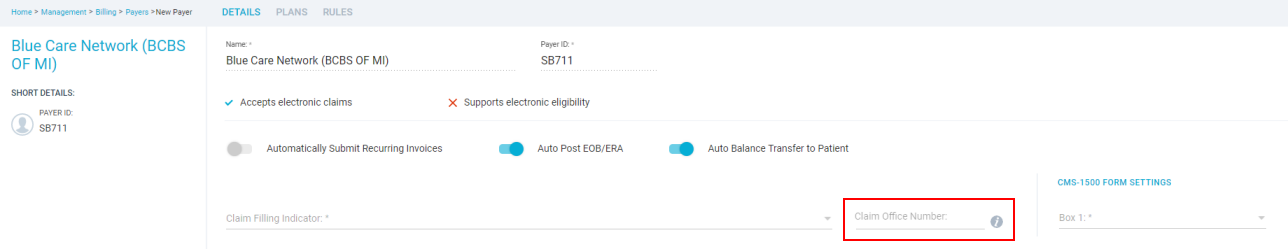This is a screenshot of a user interface with a predominantly white background. The interface features a very light blue navigation bar at the top, with sections labeled in blue font: "Home," "Management," "Billing," a section starting with "P," and "New Payer." The user has selected the "Details" tab, also in blue font.

Below the navigation bar, in blue font, the text "Blue Care Network (BCBS of MI)" is displayed prominently. Underneath, in black font, it lists "Short Details," followed by "Payer ID: 8B711." 

To the right, another section reiterates "Blue Care Network (BCBS of MI)" with "Payer ID: B8711," and it includes information about electronic claims and eligibility. There's a red "X" indicating that electronic claims are not accepted, while next to "Accepts Electronic Claims" a blue check mark shows support. 

Further down, it states "Automatically Submit Recurring Invoices," which is toggled off. Below that, "Auto Post ED6/ERA" is shown as enabled, and "Auto Balance Transfer to Patient" is also turned on.